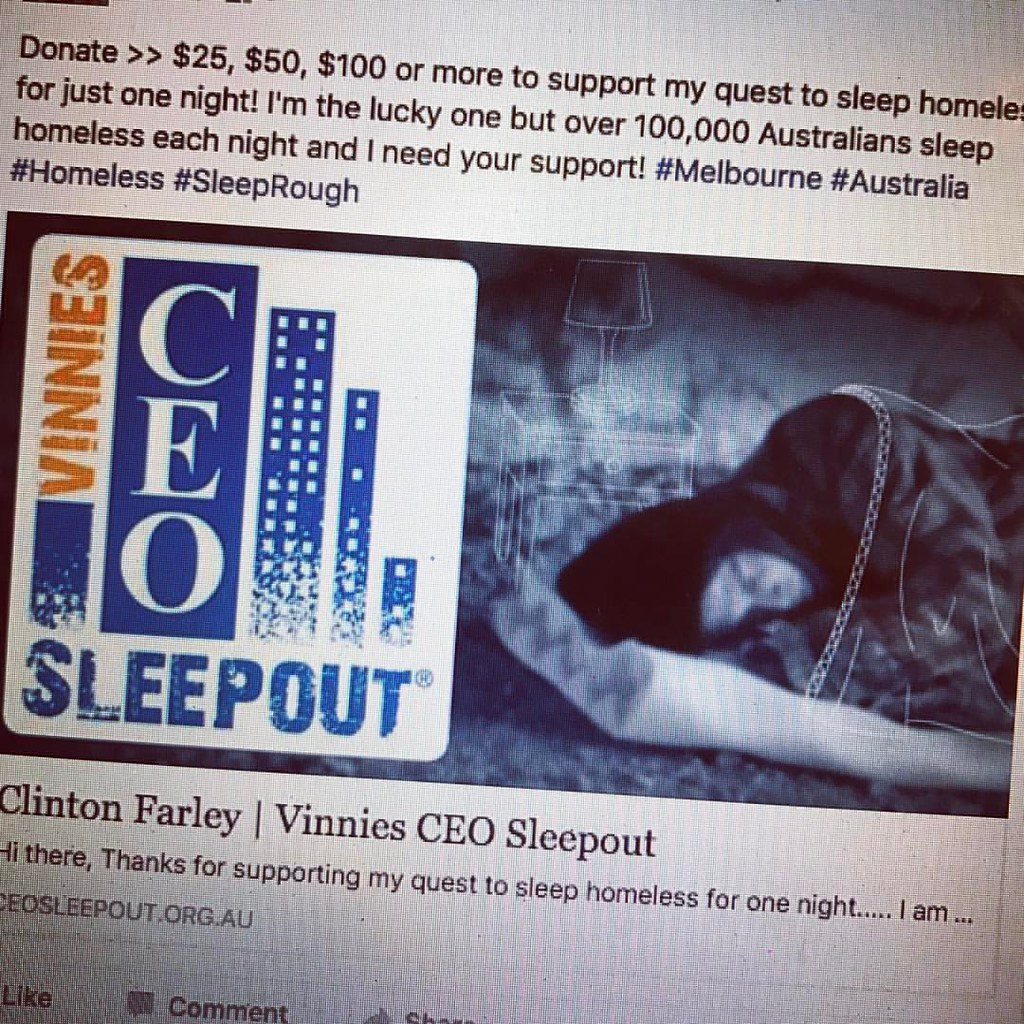The image features a photograph of an advertisement with a white background and black text. At the top, it reads, "Donate $25, $50, $100 or more to support my quest to sleep homeless for just one night. I'm the lucky one, but over 100,000 Australians sleep homeless each night, and I need your support. #Melbourne #Australia #homeless #sleeprough." Below this text, there is a black-and-white photograph of a person sleeping on a white pillow or blanket, wrapped in a black blanket, appearing to be outside. To the left of the photo, inside a white box, it says, "Vinnie's CEO Sleepout." Below this, in black text, it reads, "Clinton Farley, Vinnie's CEO Sleepout," followed by, "Hi there, thanks for supporting my quest to sleep homeless for one night," with the rest of the message cut off.